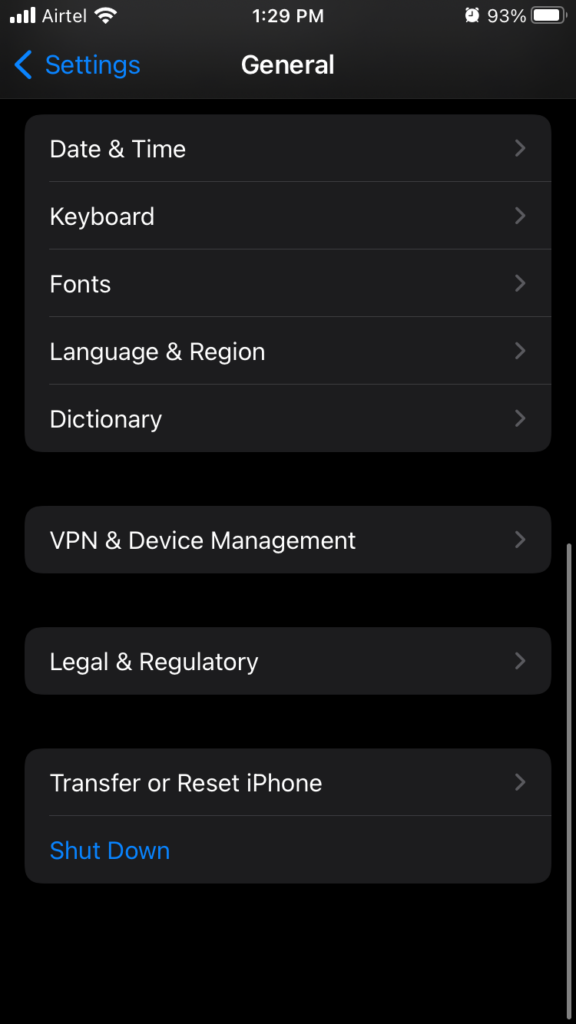The image depicts a smartphone screen in portrait mode with a dark theme. At the top left, the white text displays "Airtel," accompanied by reception and Wi-Fi symbols. In the center, the time is shown as "1:29 PM." On the top right, there is an alarm clock icon and the battery percentage "93%," along with the battery icon.

Directly below this information, a white label reads "General." To the left, in blue text, "Settings" is displayed with a left-pointing arrow. Below this, the main section of the screen features a gray background area with different settings categories separated by lines.

The first item is "Date and Time" with a right-pointing arrow, followed by "Keyboard," "Fonts," "Language and Region," and "Dictionary." The next section, labeled "One Item," includes "VPN and Device Management." Further down, "Legal and Regulatory" is listed.

At the bottom of the screen, the text "Transfer or Reset iPhone" is shown in white, with "Shutdown" written in blue text directly beneath it. The layout is clear, with each category distinctly separated and visually organized for easy navigation.